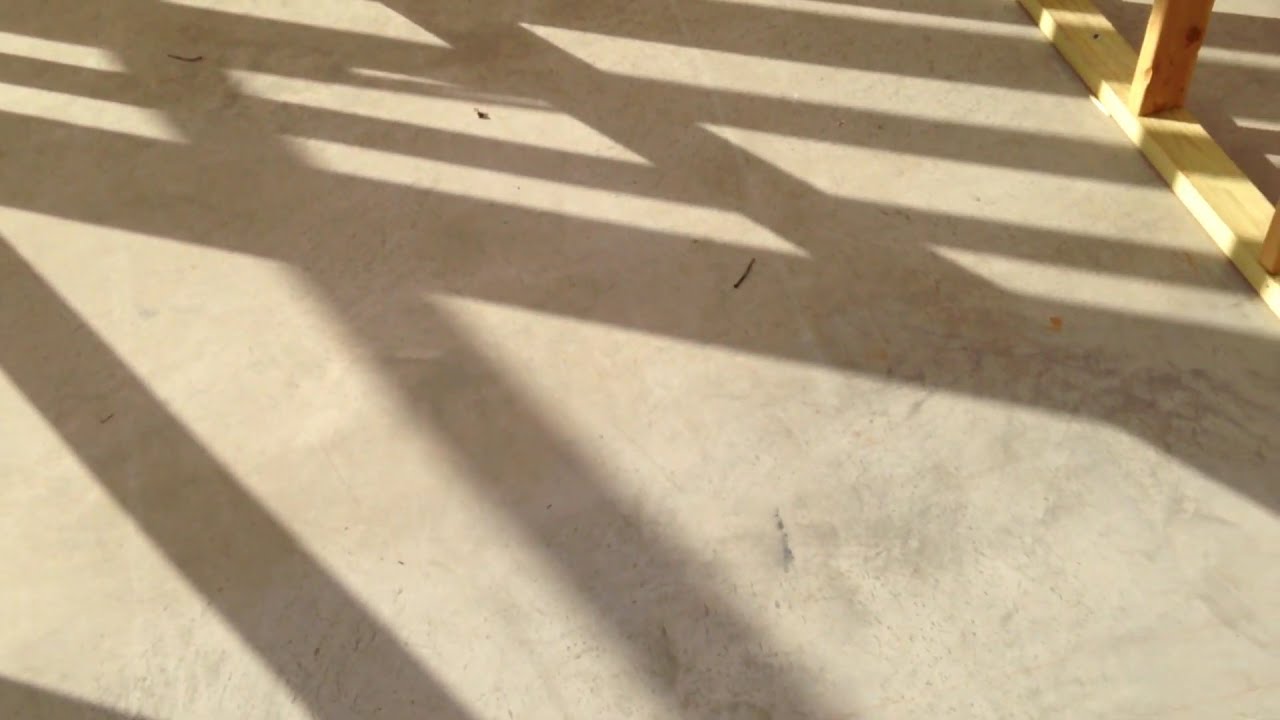This image depicts an unfinished concrete floor, likely part of a construction site. The floor appears freshly laid and is littered with small twigs and debris that seem to have been either blown in or dragged in. Dominating the visual is a complex interplay of intersecting shadows cast in various directions across the floor, suggesting the presence of multiple objects out of the frame. In the upper right corner, parts of a wooden frame are visible—their pale, bare surfaces hint at the raw, uncompleted structure of an inner wall, yet to be covered with materials like sheet rock. The only colors in the image are subtle shades of gray, tan, and brown, accentuated by patches of sunlight. The setting seems to be outdoors, under midday sunlight, adding a harsh clarity to the shadows and overall scene.